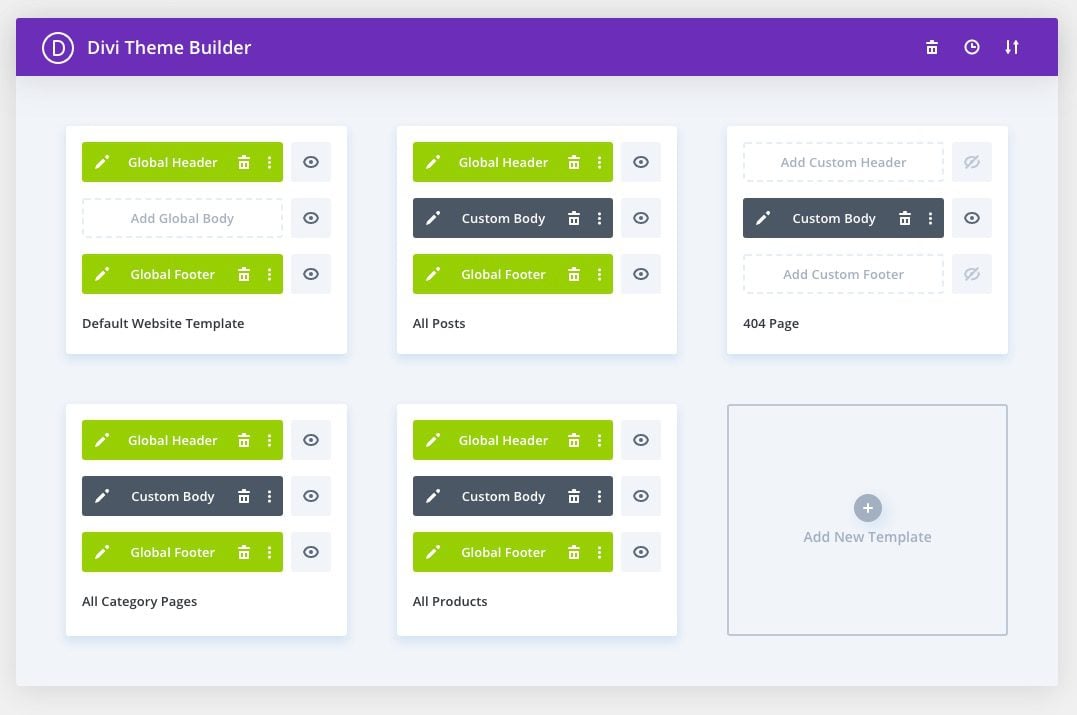The image displays a user interface of the Divi Theme Builder. At the very top, there's a dark purple border with the text "Divi Theme Builder" prominently displayed. A circular icon with a "D" in the center is placed to the left, while the top right corner features several icons: a trash can, a clock, and arrows pointing up and down.

Below this, the top left of the interface shows a white rectangular box labeled "Default Website Template," with a green box labeled "Global Footer" above it. Additionally, there is a smaller white box that says "Add Global Body."

Directly above these elements, another green box labeled "Global Header" is positioned. 

On the right side, towards the bottom, you can see the text "All Posts." Also, positioned near the bottom right, there is a green box labeled "Global Footer" followed directly by a dark blue box that says "Custom Body." 

Towards the upper part of this section, there's another green box labeled "Global Header." At the bottom right, you can see the label "404 Page," and just above this label, there's a white box that says "Add Custom Footer."